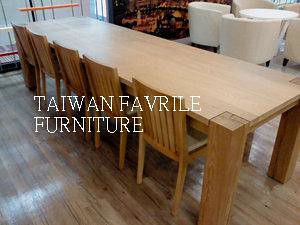The photograph showcases a furniture advertisement, prominently displaying the brand "Taiwan Favrile Furniture" in bold white text across the center. The setting features a light, wooden floor with a notable reflection, hinting at natural lighting from a large window or French doors with black edging in the top left corner. Central to the image is an extremely long rectangular dining or meeting table made of maple, extending diagonally from the top left to the bottom right. This substantial table is supported by thick, stocky legs and is accompanied by five matching wooden chairs with slatted backs, all positioned along one side of the table. In the upper right corner of the room, a cozy conversational area can be seen, consisting of four scooped low-profile chairs in a cream color arranged around a small, round white table. Adjacent to this seating arrangement is a brick fireplace, possibly containing some logs. The meticulous arrangement of the furniture and the interplay of maple and walnut tones combine to create an inviting and harmonious interior space.